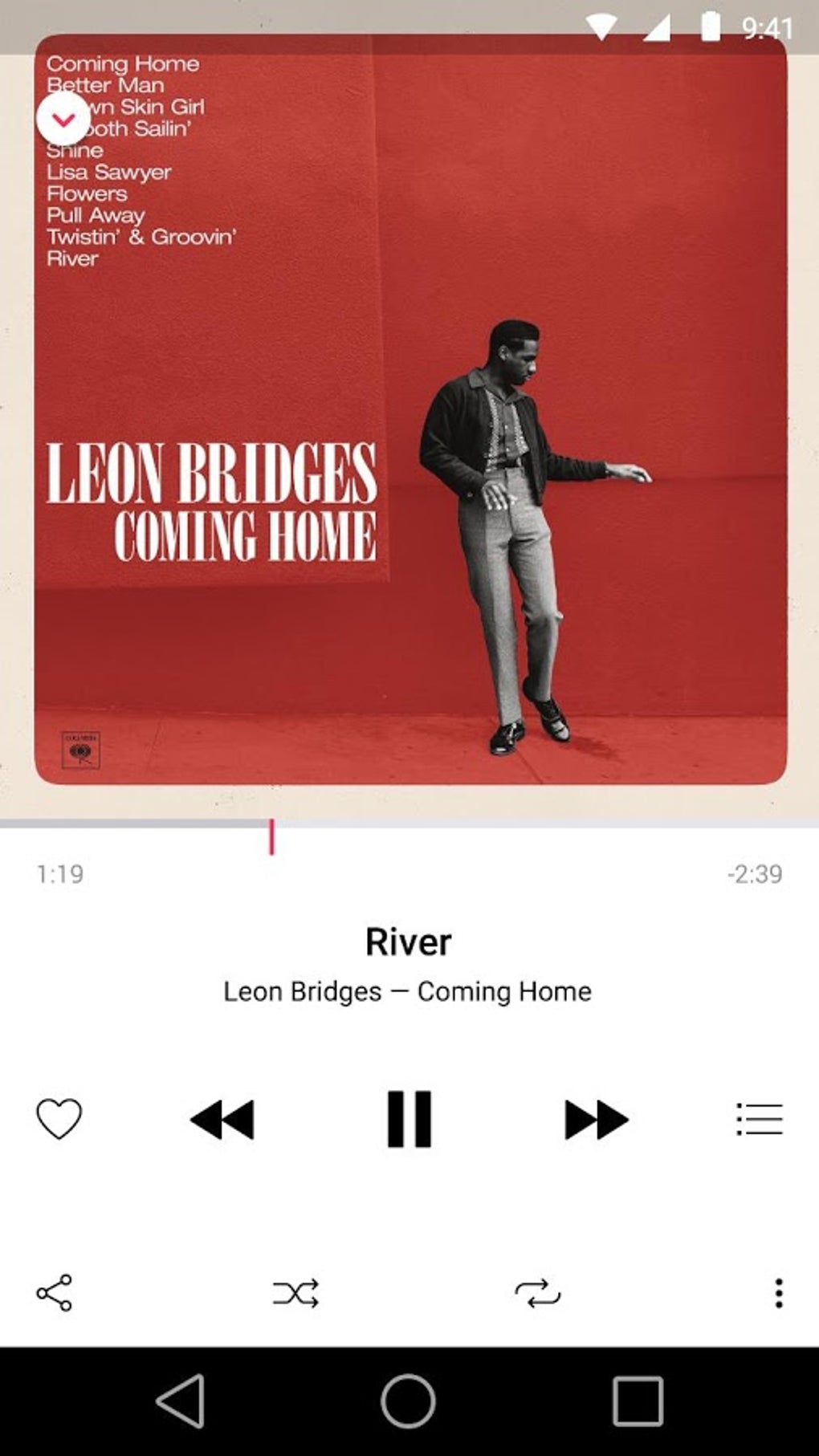This image is a screenshot of a mobile device running on Android, as indicated by the navigation bar at the bottom featuring the iconic left-facing arrow, circular home key, and square apps button unique to the Android operating system. The screenshot captures a moment from a music player app, although it is unclear if it is Spotify due to the white background—distinct from Spotify's usual dark theme. 

The player controls at the bottom are black, with the pause button prominently highlighted, indicating the song is currently paused. The interface features a clean, white background with black text and controls, giving it a minimalist aesthetic.

Dominating the screenshot is the album cover art for "Coming Home" by Leon Bridges. The cover art consists of a square image with a light tan border framing a striking red interior. The scene within depicts a black-and-white photograph of Leon Bridges, a black man leaning casually against the red wall. He appears to be wearing brown or gray pants, though the black-and-white nature of the photo makes it difficult to discern the exact color.

Prominently displayed in large white block letters next to him are the words "Leon Bridges Coming Home." In the upper left-hand corner, the tracklist is listed in white text against the red background. At the moment captured in the screenshot, the song "River" is playing at 1 minute and 19 seconds, with 2 minutes and 39 seconds remaining.